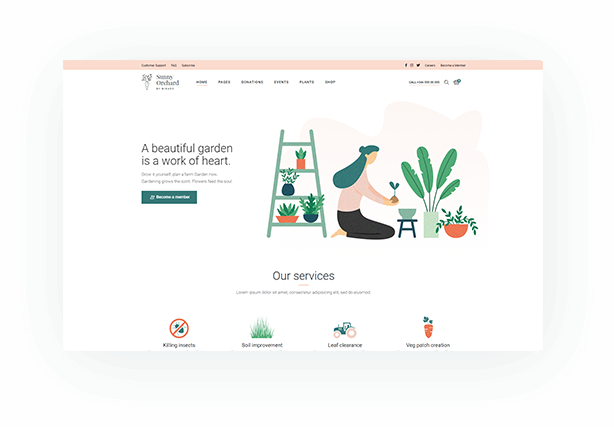The landscape-oriented screenshot features a white background with a serene, digitally created illustration at its center. A woman, depicted kneeling and facing to the right, is tenderly placing a plant into a pot, surrounded by multiple plants, including four displayed on a ladder. Above the illustration, the text "A beautiful garden is a work of art" adds a poetic touch. Below the woman, the phrase "Our Services" introduces the lower section which is lined with four icons and corresponding phrases: "Killing Insects," "Soil Improvement," "Leaf Clearance," and "Vegetable Patch Creation." The muted greens and pops of orange throughout the design create a cohesive and aesthetically pleasing palette. Additionally, the top of the screenshot features a light bar with some blurred text, adding to the overall composition.